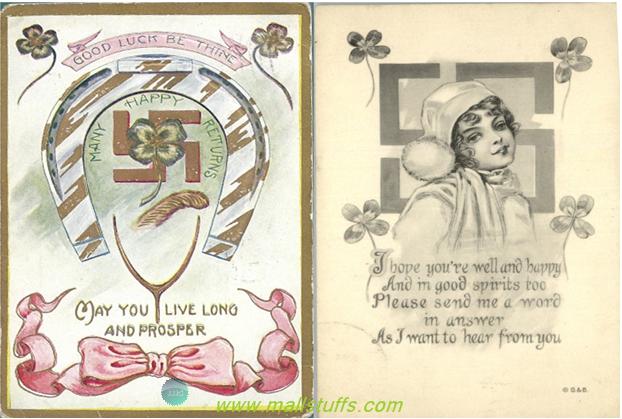The image appears to be an old, possibly vintage card, divided into two panels. The left panel serves as the cover and is set against a white background. At the top, it features two four-leaf clovers, one positioned on each side, encased within a yellow or gold banner. Just beneath this, there is a white and brown horseshoe with a pink banner draped over it, bearing the words "Good luck be thine" in black letters. The interior of the horseshoe displays the phrase "Many happy returns," and directly below it rests a swastika symbol interwoven with another four-leaf clover. Further down, a wishbone appears, accompanied by the phrase "May you live long and prosper." The bottom of this panel is adorned with a pink bow, from which ribbons curl elegantly upward on each side.

The right panel seems to be the card's interior and features a beige background. It showcases a black-and-white illustration of a young girl wearing what appears to be a nightgown and a stocking cap with a large ball at its end. Four four-leaf clovers, two on each side, frame the girl. Below her image, the text reads, "I hope you're well and happy, and I'm in good spirits too. Please send me a word and answer as I want to hear from you." This detailed old card combines elements of luck and well-wishing, punctuated with vibrant illustrations and heartfelt messages.